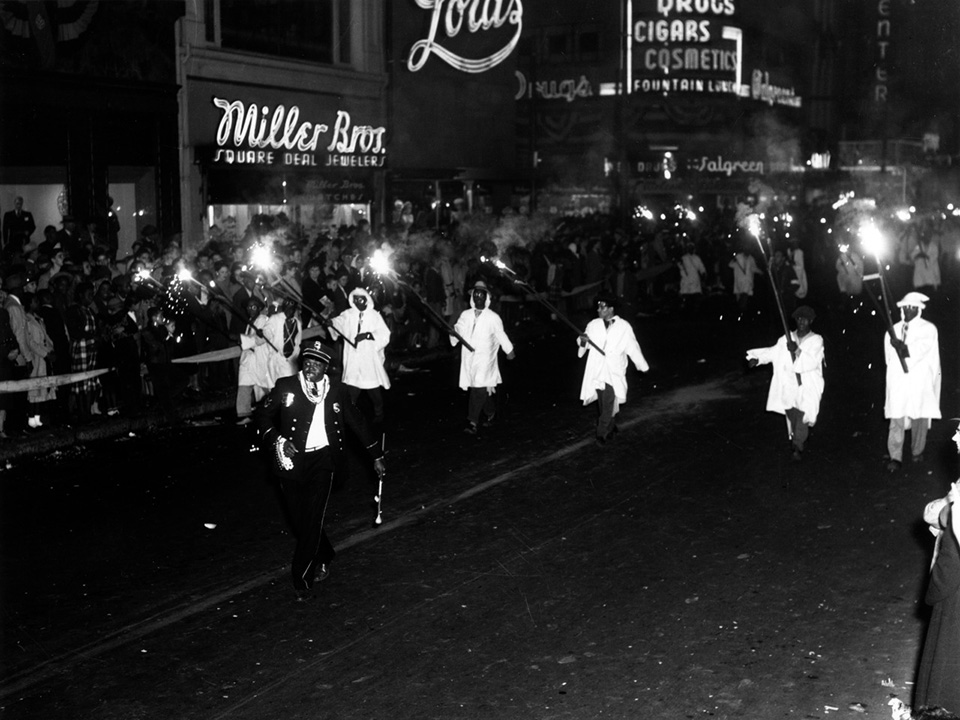The black-and-white vintage photograph captures a nighttime street scene during what appears to be a parade. In this landscape-oriented image, a black man dressed in a police-style band uniform—with a hat and baton—leads the march, moving towards the bottom left corner. Behind him is a row of six individuals dressed in white overcoats or hooded robes, all carrying torches that illuminate the scene. The background shows several out-of-focus individuals also in white coats. Spectators crowd the left sidewalk, held back by a white ribbon, while flashing camera lights add to the atmosphere.

The parade proceeds past store signs that read "Miller Brothers" and "Walgreens." Another store sign, in cursive, identifies the "Miller Bros Square Deal Jewelers." Another shop advertises "Cigars, Cosmetics." This bustling night scene, filled with the glow of neon signs and torches, is a faithful representation of a historic city street parade.